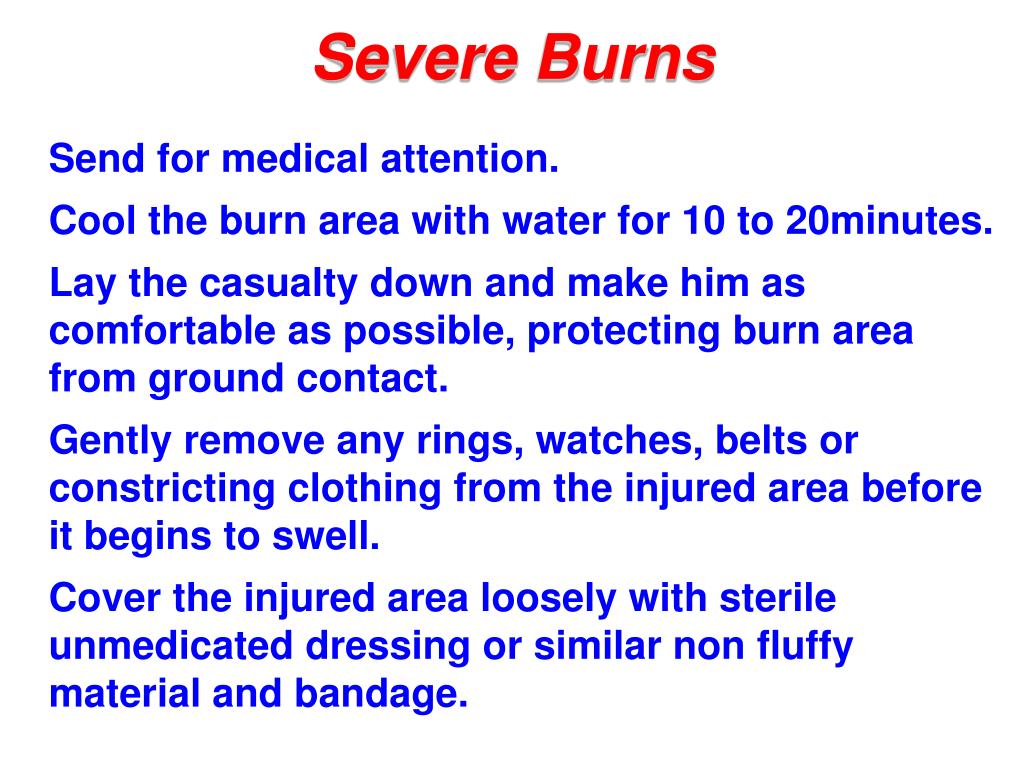In the center-top of the white background image, a red italicized heading reads "Severe Burns." Below this heading, there are detailed first-aid instructions in blue, left-justified text, organized into five main points. The first point advises to "Send for medical attention." The second point instructs to "Cool the burn area with water for 10 to 20 minutes." The third point states, "Lay the casualty down and make him as comfortable as possible, protecting the burn area from ground contact." The fourth point recommends, "Gently remove any rings, watches, belts, or constricting clothing from the injured area before it begins to swell." The final point advises to "Cover the injured area loosely with sterile, unmedicated dressing or similar non-fluffy material and bandage." This text provides essential first aid steps for treating severe burns.